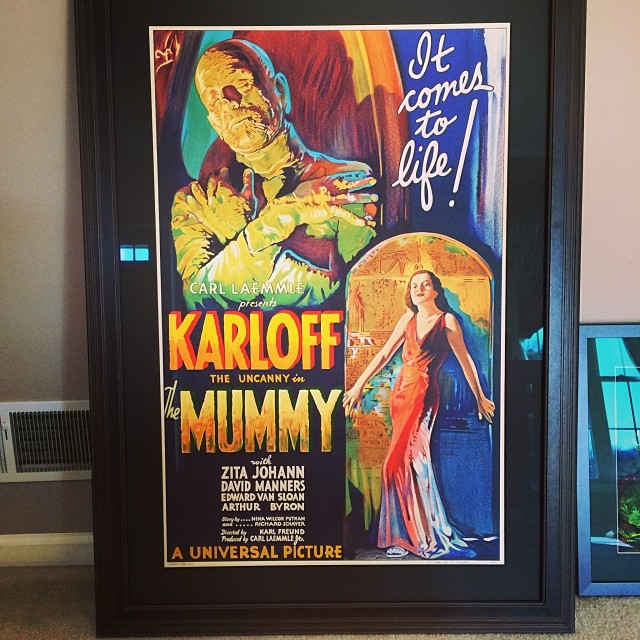This is a detailed photograph of a framed movie poster for the film "The Mummy," set indoors with a gray wall and a window to the right. The poster itself is vertical and set in a black frame with a black mat. It features a rich palette of reds, blues, yellows, and whites. In the upper-left corner, there is a photorealistic graphic of a mummy with its arms crossed over its chest and hands near its shoulders. To the right of this mummy image, the text reads, "It Comes to Life!" in cursive. Below this, in a box with additional text, it says, "Carl Laemmle presents Karloff, the Uncanny, in The Mummy, with Zita Johann, David Manners, Edward Van Sloan, and Arthur Byron. A Universal Picture." On the left side of the poster is a vertical statement with further credits, including a story by Nina Wilcox Putnam and Richard Schayer, produced and directed by Karl Freund, and produced by Carl Laemmle Jr. In the bottom-right section of the poster, there is a graphic of a woman, depicted as a white woman, wearing a low-cut, long red evening gown. She stands with her knee bent and arms outstretched, leaning against a wall that appears to have hieroglyphics on it.